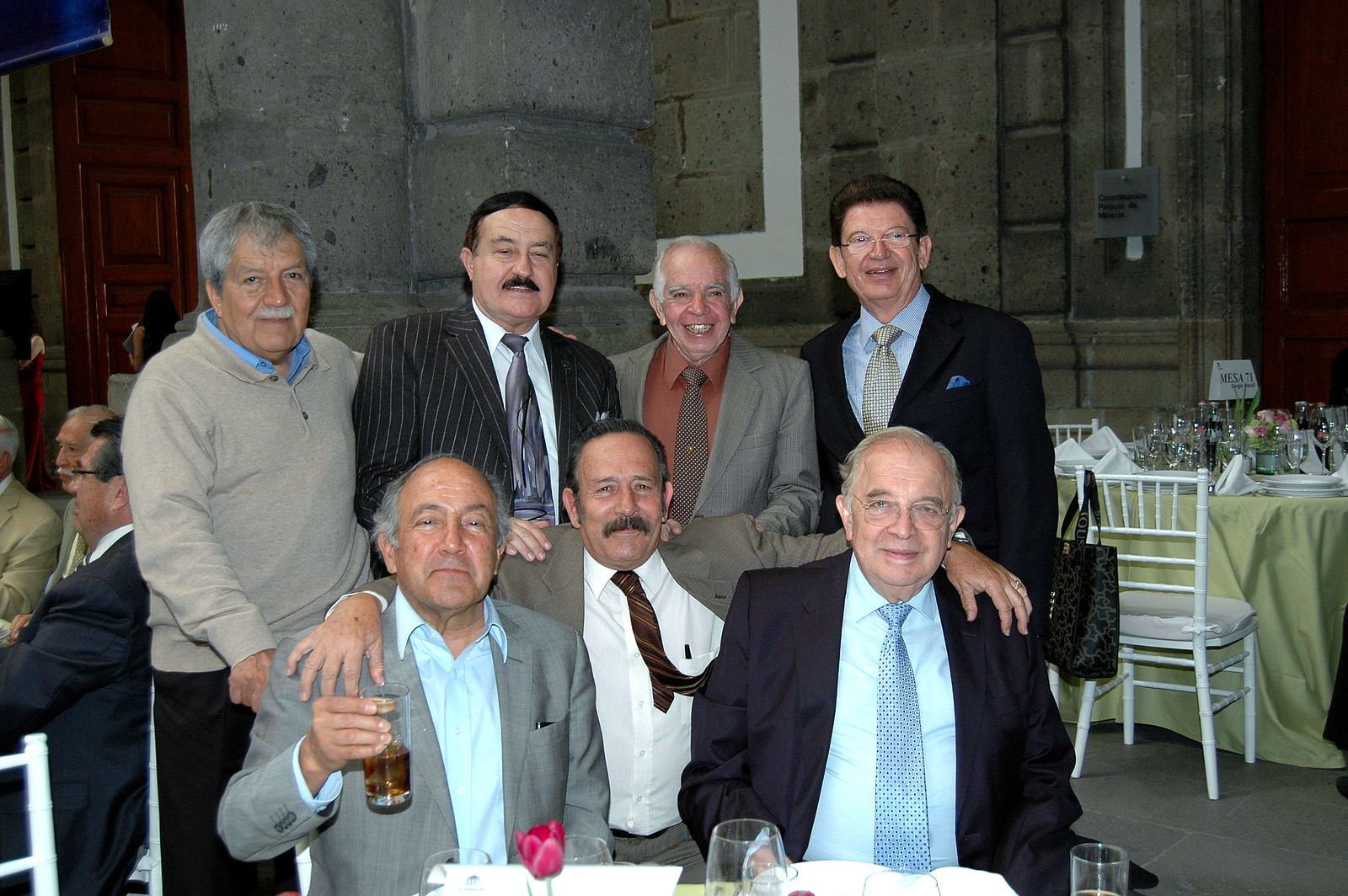This photo captures a reunion of seven older Caucasian gentlemen, most likely long-time friends, likely in their late 40s to early 60s, gathered together in a well-lit banquet setting. All of them are dressed in formal or semi-formal attire, with five donning ties. Three gentlemen are seated in the front row, with the man on the left holding a beer, dressed in a grey sport jacket and white dress shirt. The middle gentleman, characterized by his blackish hair and mustache, has his arms around the other two; he is wearing a grey sport coat, white jacket, and a red and black striped tie. The gentleman on the far right is smiling, sporting grey hair, a black sport jacket, a white dress shirt, and a pink tie.

Standing behind them are four men, all smiling at the camera. They include a gentleman with grey hair, a grey sweater, and black pants, another with black hair and a black mustache dressed in a black striped suit jacket, a third with grey hair, bald on top, wearing a grey coat and a reddish dress shirt with a green tie, and lastly, a man with black hair and glasses, in a black suit with a white shirt and a cream-colored tie.

In the background, on the right side, there is a banquet table covered with a greenish tablecloth and set with tableware. To the rear left, some other attendees are partially visible, sitting at a table. The setting further includes architectural elements like a big brown door on the left, a dark black door on the upper right, a large grey stone pillar, and a blue banner hanging in the upper left. This detailed scene where old friends reconnect showcases their enduring camaraderie.